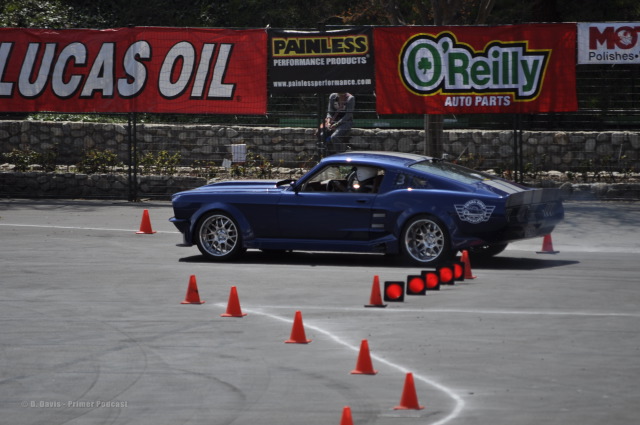An outdoor image depicts a vintage royal blue Mustang fastback navigating an obstacle course marked by around 12 to 15 small orange cones. Several cones are knocked over, suggesting the car might have strayed slightly from the intended path. The Mustang is centered in the frame, occupying roughly 20% of the image height and 60% of its width, with a person wearing a white helmet at the wheel. The car is oriented towards the 9 o'clock position against a backdrop of a sunny, paved area. Prominent in the background, hanging on a fence, are a series of colorful banners. One banner advertises Lucas Oil with white letters on a red background. Another highlights Painless Performance Products, featuring black letters on a yellow background and white letters on a black background. There's also a banner for O'Reilly Auto Parts, distinguished by its green lettering and shamrock logo. An additional, less clear banner mentions M.O. and some products related to polishes. The overall scene is dominated by the vibrant blue of the Mustang contrasted against a gray asphalt track under bright lighting.